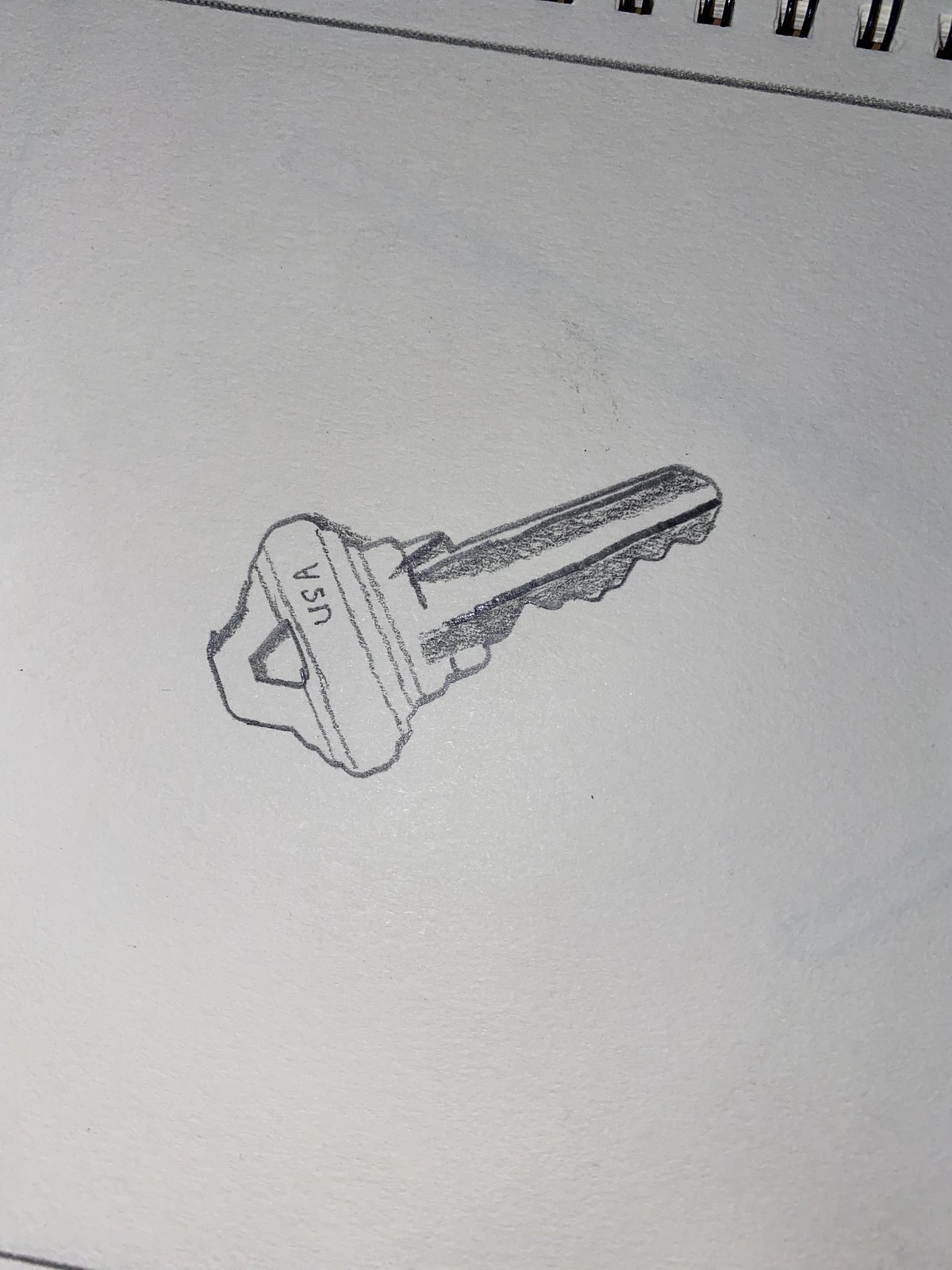The image showcases a detailed pencil sketch of a key on a sheet of paper from a spiral-bound sketch pad, as indicated by the black spirals visible in the top right-hand corner. The sheet appears to have a hand-drawn diagonal line extending across the top portion and a similar line in the bottom left-hand corner, adding a textured background to the drawing.

The key itself, rendered in fine pencil work, features a standard design. The head of the key prominently displays the text "USA," along with horizontal striping for added detail. The topmost part of the key includes a triangular section, completing the classic key shape. Moving downward, the shaft of the key—the part that would be inserted into a lock—is meticulously shaded. This section tapers off into a jagged, bumpy edge with slight curves, portraying the intricate notches that are characteristic of keys used in locks. The precise pencil work and shading suggest that the key may have been initially traced and subsequently filled in to enhance its realism.